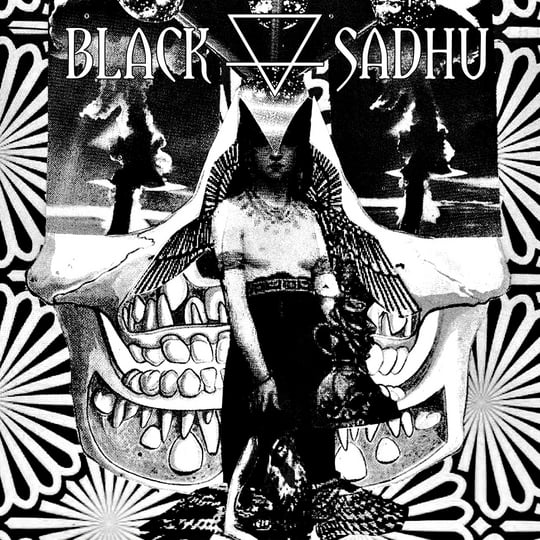This black and white image, evocative of an old vinyl or CD cover, prominently features the title "Black Sadhu" in white letters at the top. Between "Black" and "Sadhu" is an upside-down pyramid outlined in white, with a horizontal line dissecting its lower third. Beneath this emblem is a striking human figure adorned with black and white wings. The figure appears to be a woman wearing a white, high-waisted skirt with a prominent belt, and her chest is bare, with shadows accentuating her breasts. An ornate necklace adorns her neck, and she holds an artifact in each hand.

Her head is covered by a silver, triangular headdress that narrows down to her nose and flares outward as it ascends, flowing dramatically to either side of her head. Surrounding her head on both sides are backlit mushroom clouds, adding to the surreal and intense atmosphere.

The backdrop behind her is a series of detailed, sharp teeth-like structures, giving the impression of a monstrous maw. Accompanying this elaborate scene are black and white flowers or psychedelic designs, further enhancing the image's otherworldly and graphic quality.